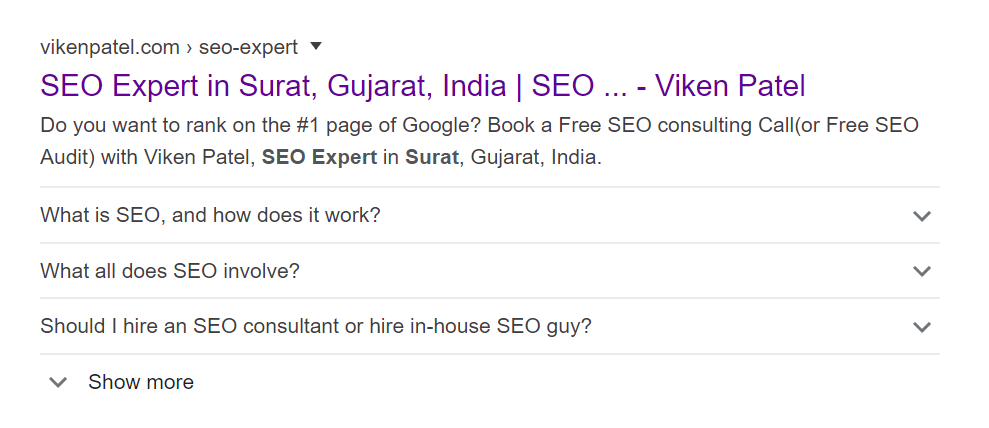The image features text on a white background and is an advertisement for an SEO expert. At the top, the website "BeaconPatel.com" is prominently displayed. Below it, in purple text, a clickable link reads "SEO Expert in Surat, Gujarat, India. SEO Beacon Patel."

Further down, there is a compelling offer: "Do you want to rank on the number one page of Google? Book a free SEO consulting call or free SEO audit with Beacon Patel, SEO expert in Surat, Gujarat, India."

Next, there are three expandable questions with downward-pointing arrowheads next to each one:
1. "What is SEO and how does it work?"
2. "What all does SEO involve?"
3. "Shall I hire an SEO consultant or hire an in-house SEO guy?"

At the bottom, the text "show more" also features an expandable arrowhead, indicating additional information is available.